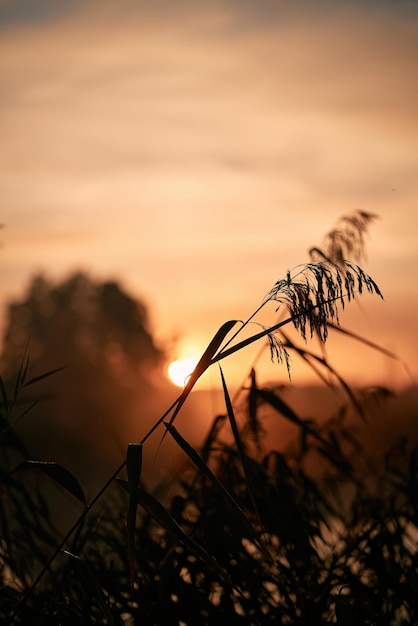A serene nature scene captures the first light of dawn. In the foreground, a prominent tall blade of grass rises gracefully to the right, surrounded by an overgrowth of wild grasses. Some additional grasses edge off slightly out of the frame, blending into the composition. The background showcases a blurry, yet radiant, sunrise centrally positioned, with the sun casting a soft glow. To the left, a large tree with dense, bushy foliage stands slightly out of focus. The sky above is adorned with white, fluffy clouds, tinged with a hint of blue at the top. As the sun peers through the tall grass, a pinkish-orange hue paints the horizon, blending seamlessly into the ethereal, blurred backdrop.